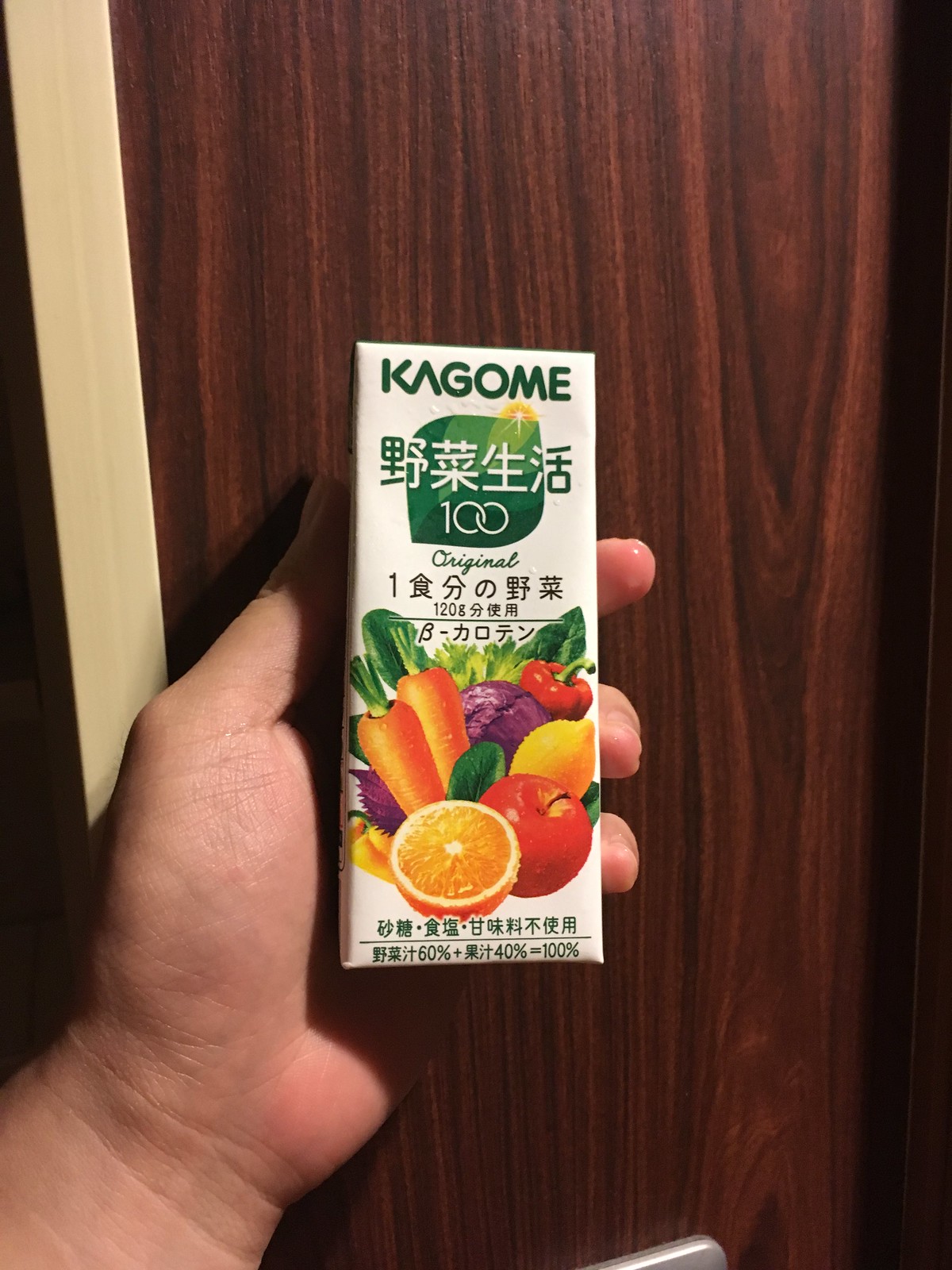In this detailed photograph, a person is seen holding a white box of juice. The individual’s hand is emerging from the bottom left corner of the image, firmly grasping the box. The background includes a brown door, which adds a subtle, contrasting backdrop to the vibrant packaging of the juice. 

The top part of the juice box features a white section with green accents, prominently displaying the brand name "Kagome." Below this, there is Japanese lettering, accompanied by the phrase "100 original." The lower portion of the box is richly illustrated with various colorful graphics. These graphics include images of orange carrots with green leaves, vibrant green lettuce, a purple head of cabbage, a red pepper, a yellow lemon, a red apple, and a neatly sliced open orange. At the very bottom of the box, more text, likely in Chinese, can be seen, adding to the international appeal and authenticity of the product.

The overall composition of the photograph provides a comprehensive view of the juice box, highlighting its brand, ingredients, and multilingual labeling against a simple yet effective background.